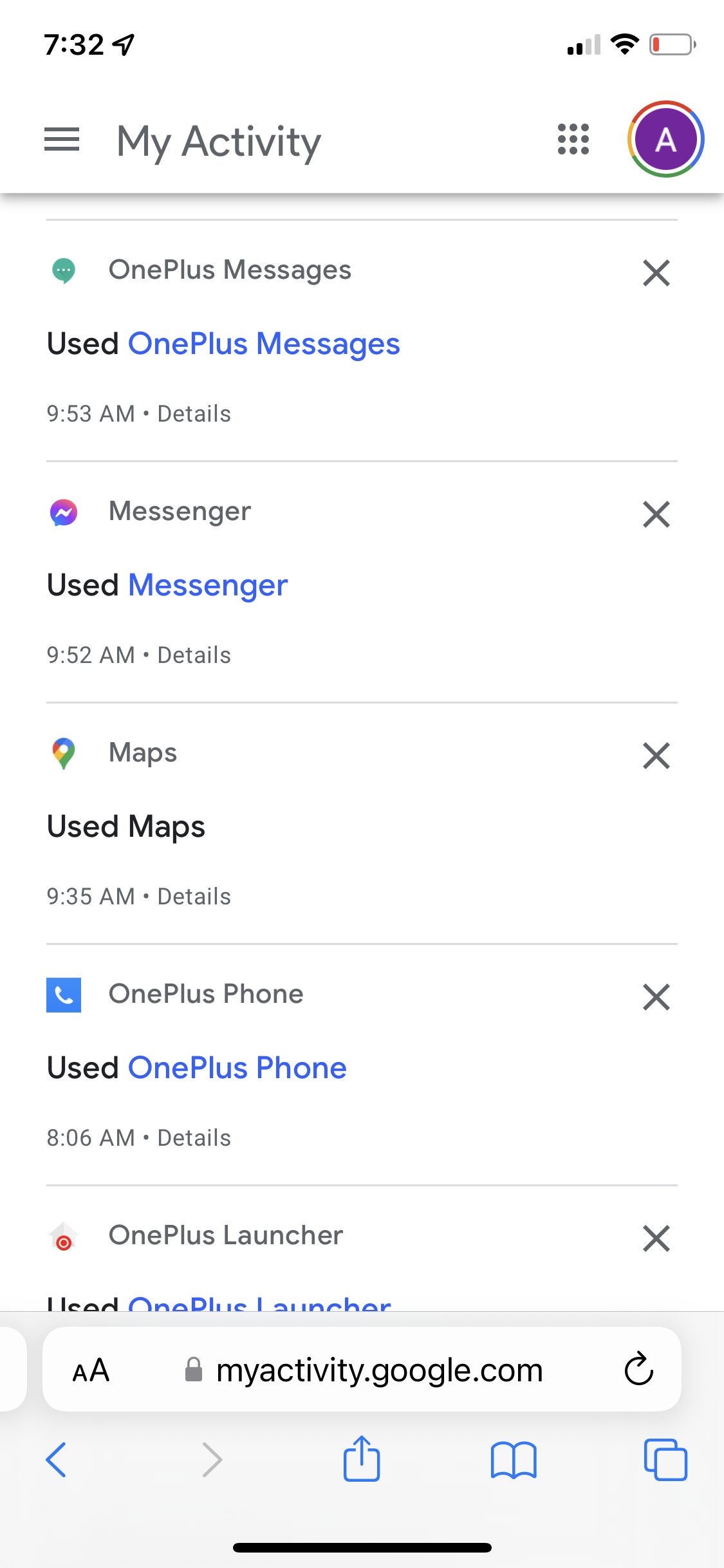This image is a screenshot from a smartphone with a white background, showcasing the "My Activity" page on a Google account. The top left corner displays the time as 7:32, without specifying a.m. or p.m. On the top right, icons for the battery (which is almost drained), Wi-Fi, and wireless connections are visible. Below this, on the left side, the text "My Activity" appears next to three horizontal lines indicating a menu. On the right side, a purple circle with the letter "A" likely represents the user's Google account avatar.

A gray line separates the header from the main content. The main content consists of a list of recent activities with corresponding icons and descriptions. Each item has a gray "X" on the right side, possibly for deletion. The list includes:

1. **OnePlus Messages** – with the phrase "Used OnePlus Messages" in blue.
2. **Messenger (Facebook Messenger)** – with the Messenger icon and the text "Used Messenger."
3. **Maps (Google Maps)** – with the Google Maps icon and the text "Used Maps."
4. **OnePlus Phone** – displayed with a blue square icon containing a white phone and the text "Used OnePlus Phone."
5. **OnePlus Launcher** (at the bottom) – although not elaborated in the provided content, it is listed among the activities.

At the very bottom of the screenshot, the web address "myactivity.google.com" is shown.